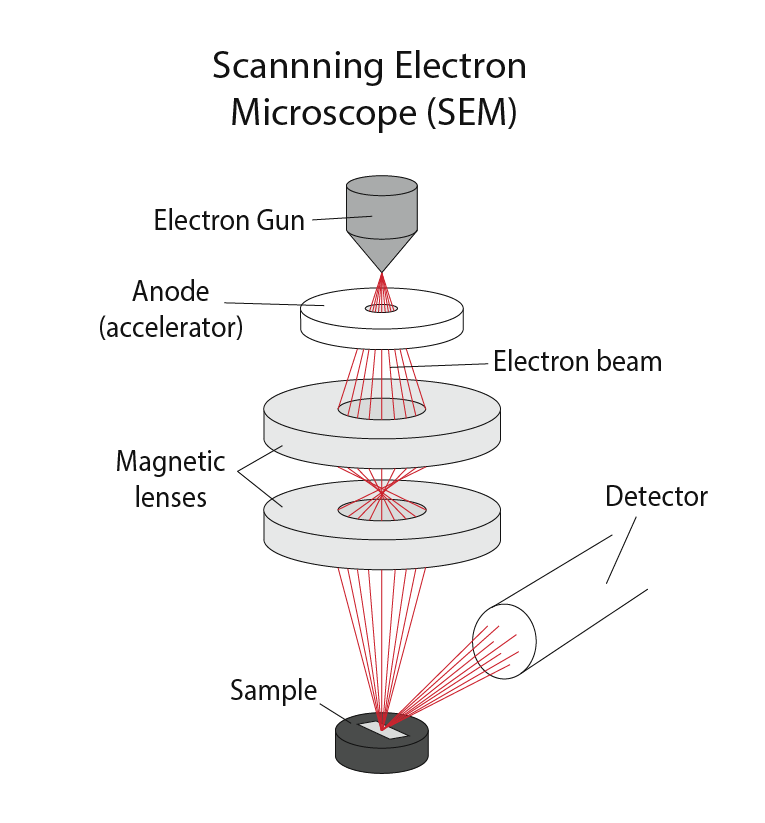The image is a detailed diagram of a Scanning Electron Microscope (SEM). At the top of the device, there's a gray cylinder labeled "Electron Gun," from which red electron beams are emitted. These beams are directed through a white cylindrical component called the "Anode Accelerator," which has a hole in the center. The diagram shows these beams emerging in a circular pattern and passing through two gray disks labeled "Magnetic Lenses." Here, the beams converge and focus to a single point before hitting the "Sample," placed below the lenses. Next to this setup is a long cylindrical pipe labeled "Detector." The image uses red lines to illustrate the electron beam's path and employs light and dark gray shades for the components, all set against a white background.